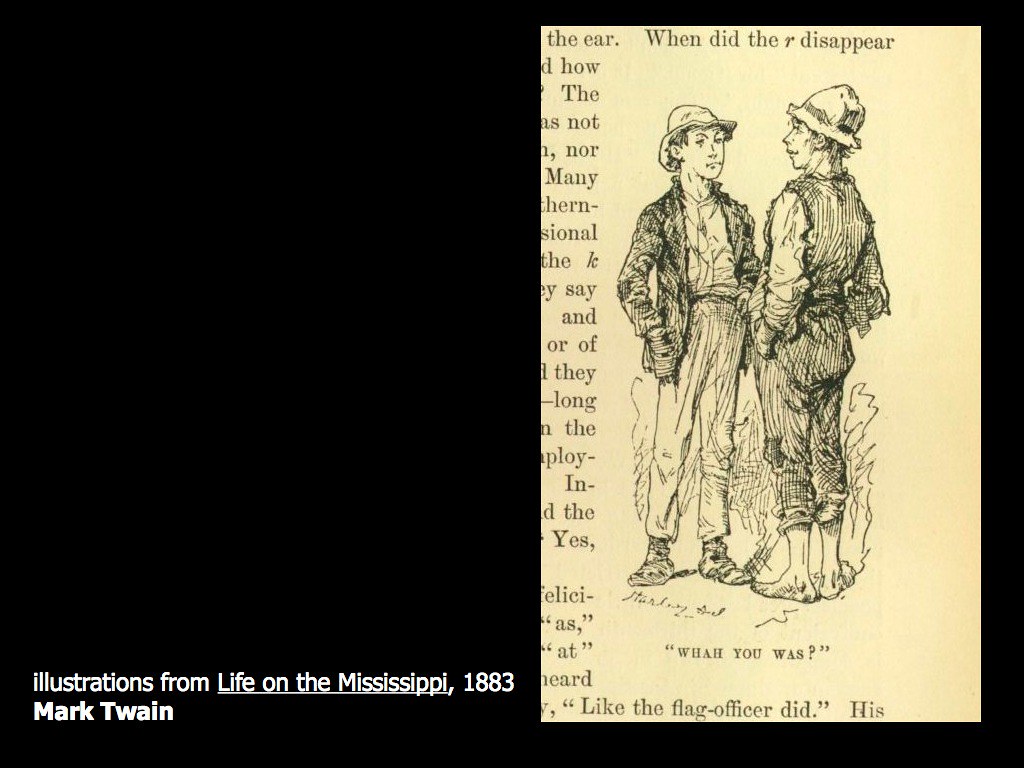The image features a black background with a balanced layout. The left half of the image is predominantly empty, except for some white text at the bottom that reads, "Illustrations from Life on the Mississippi, 1883, Mark Twain." This white text provides a historical context for the content depicted on the right. 

The right half showcases an illustrated page from a book. The page has a light brown hue and features an intricately detailed pencil drawing of two young boys, possibly representing Huckleberry Finn and Tom Sawyer. One boy is dressed in a rumpled suit coat, long pants, and shoes, while the other wears a striped vest and pants, and is barefoot. Both boys appear to have felt crush hats on their heads. The drawing is surrounded by partially visible text on the page. At the bottom of the drawing is a phrase that reads, "for you?" 

The entire composition is neatly framed within a black rectangular border, accentuating the historical and literary significance of the illustration.